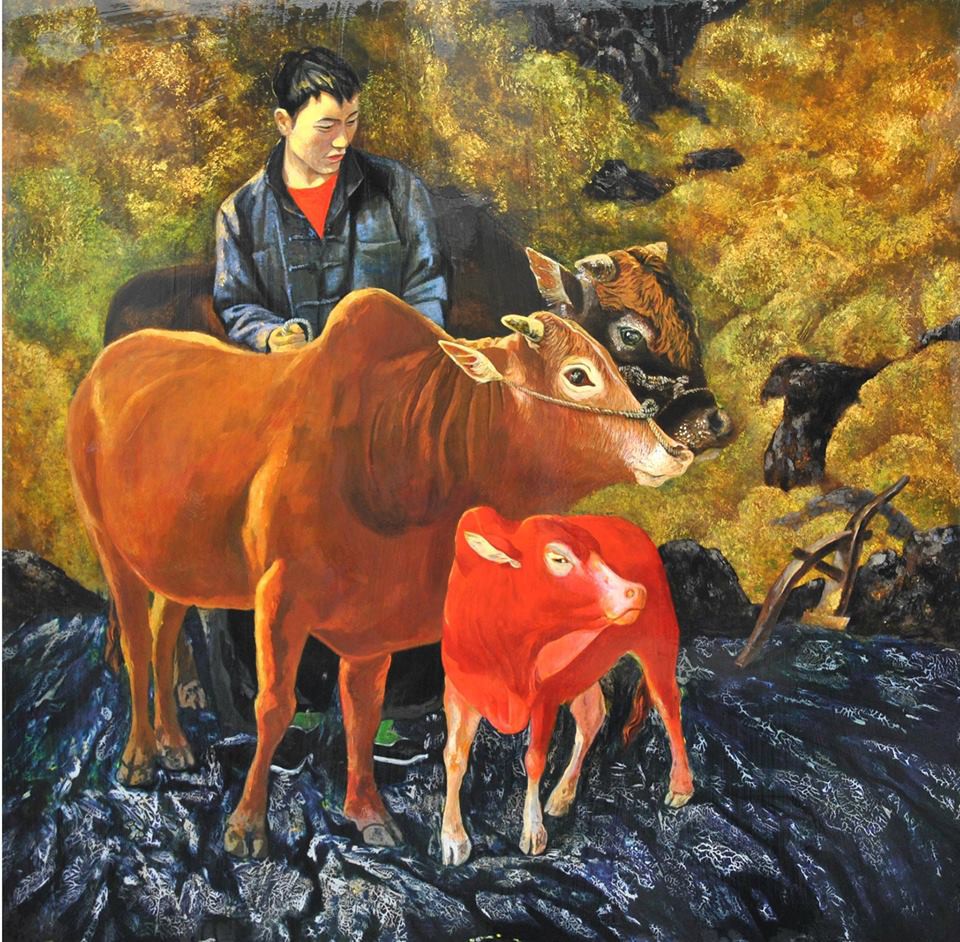This painting depicts a young Asian man standing between a group of cows on a shiny, volcanic-like, black rocky ground. The man, who has short black hair, is wearing a blue denim-like over shirt with a red shirt underneath. To his sides are two large cows, with one cow displaying a golden brown hue with short horns, and the other being a dark brown with some brown patches and short horns as well, each adorned with gray rope bridles around their faces. In front of these two cows stands a small, bright reddish-brown calf with a bit of white on its legs. The scene is set against a backdrop of golden, almost whimsical, tree-like shapes or shrubs, painted with bright, speckled strokes.